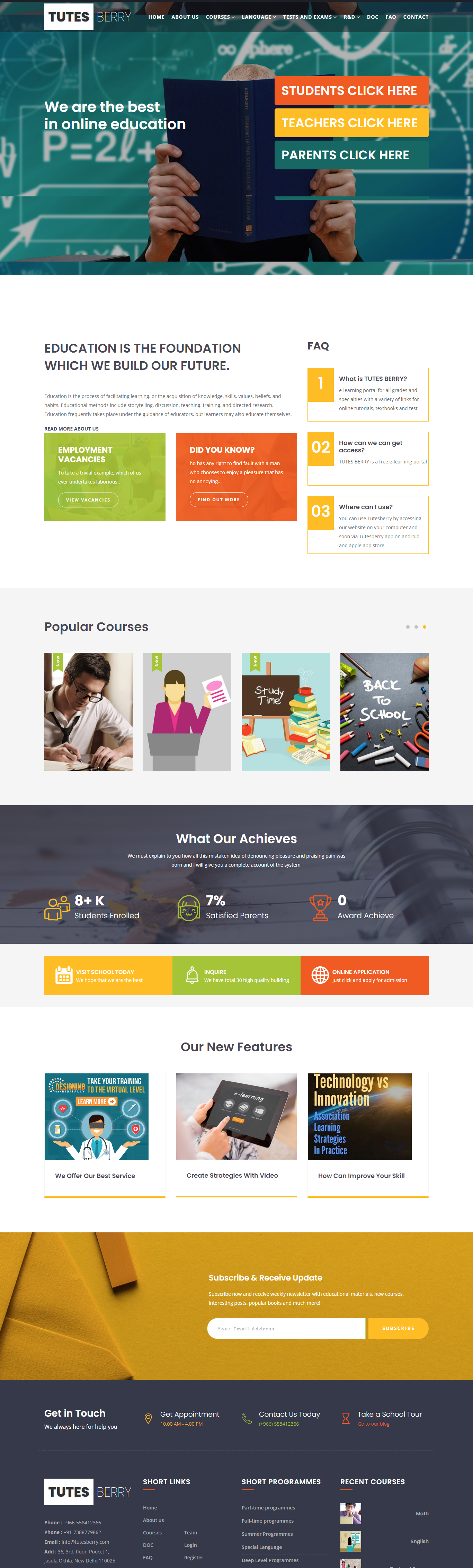Certainly! Here is a cleaned-up and detailed caption for the described image:

---

The image showcases an introductory splash page for a company named Tootsberry. The logo and brand name "Tootsberry" are prominently displayed in the upper left-hand corner. The navigation menu spans across the top, featuring tabs labeled as follows: Home, About Us, Courses (with a drop-down menu), Language (with a drop-down), Tests and Exams (with a drop-down), R&D (with a drop-down), Doc, Fac, and Contact.

The background features a green chalkboard filled with various equations and small mathematical diagrams. Overlaying the background, white text on the left side reads, "We are the best in online education." On the right side, three brightly colored call-to-action boxes are visible: an orange box labeled "Students click here," a yellow box labeled "Teachers click here," and a green box labeled "Parents click here."

Center stage is a striking but slightly distorted image of a person holding a blue book with gold writing on its spine. The image appears to be manipulated such that the person seems to have seven fingers on each hand.

Below this image, a dense block of text in smaller print reads: "Education is the foundation upon which we build our future. Education is the process of facilitating learning, or the acquisition of knowledge, skills, values, beliefs, and habits. Educational methods include storytelling, discussion, teaching, training, and directed research. Education frequently takes place under the guidance of educators, but learners may also educate themselves." Following this, a prompt reads, "Read more about us."

Additionally, a green box with the words "Employment vacancies" catches the eye. It precedes a snippet filled with filler text: "To take a trivial example, which of us ever undertakes laborious …" and ends with a call to action, "View vacancies."

On the right side of the page, an orange box labeled "Did you know?" contains another block of placeholder text: "Who has any right to find fault with a man who chooses to enjoy a pleasure that has no annoying …?" followed by "Find out more."

A series of vertical boxes labeled "FAC" on the right provide some FAQs, although the grammar is off:
1. "What is Tootsberry?" states it is "an e-learning portal for all grades and specialties, with a variety of links for online tutorials, textbooks, and tests."
2. "02. How can we get access?" explains that "Tootsberry is a free e-learning portal."
3. "03. Where can I use?" mentions that Tootsberry can be accessed via their website and will soon be available on the Android and Apple App Store.

At the bottom, four images titled "Popular courses" are shown. The first depicts a real person, the second an avatar, and the last two tags read "study time" and "back to school."

Below this section, a poorly worded heading "What our achieves" introduces a jumbled passage: "We must explain to you how all of this, how all this mistaken idea of denouncing pleasure and praising pain was born. And I will give you a complete account of the system."

Subsequent figures are listed: "8+ K students enrolled," "7% satisfied parents," and "0 awards achieved."

The final portions of the page state: 
- "With school today, we hope that we are the best. Inquire."
- "We have a total of 30 high-quality buildings."
- "Online application: Just click and apply for admission."

Finally, the section "Our new features" includes: "We offer our best service," "We create strategies with video," and "How can we improve your skill?"

Overall, the page presents a cluttered and somewhat grammatically inconsistent depiction of Tootsberry, an online educational platform, with a variety of call-to-action elements and information sections needing refinement.

---